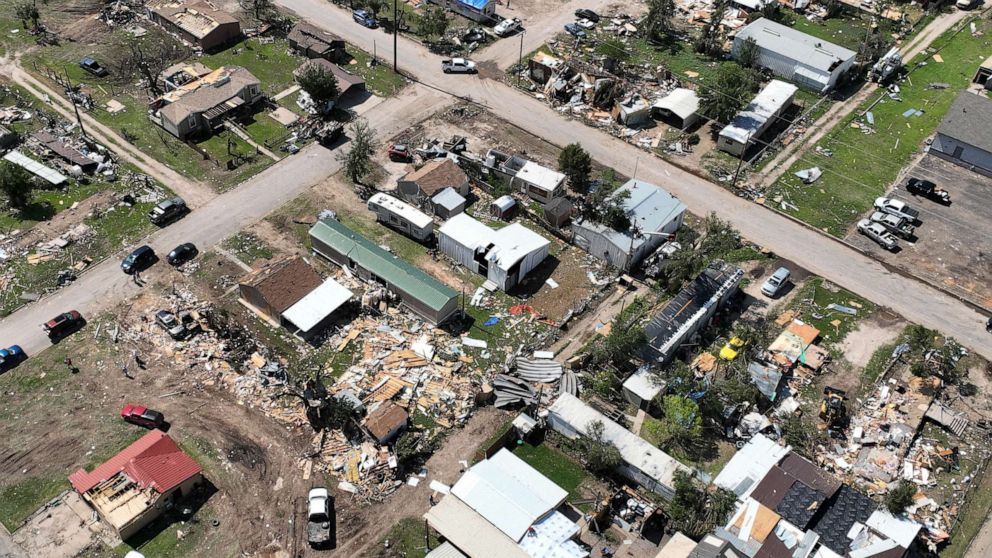This aerial view photograph captures the aftermath of a devastating event, likely a tornado, that has ripped through a community in a small town. The image, taken during the daytime at a slight downward angle, shows an intersection surrounded by multiple buildings, including homes and sheds. Some structures have been completely demolished, reduced to mere piles of rubble resembling matchsticks, while others have suffered partial roof and side damage. Debris, including twisted metal, tin sheets, and various unidentifiable items, is strewn across green lawns and bare dirt. A red building towards the bottom left stands with its roof partially torn off, indicative of the widespread destruction. Vehicles can be seen parked on streets and in alleys, underscoring the community's former normalcy. Fences and some trees remain standing amidst the chaos, illustrating the randomness of the destruction. The scene poignantly highlights significant property loss, leaving one to feel profound sympathy for the affected residents.